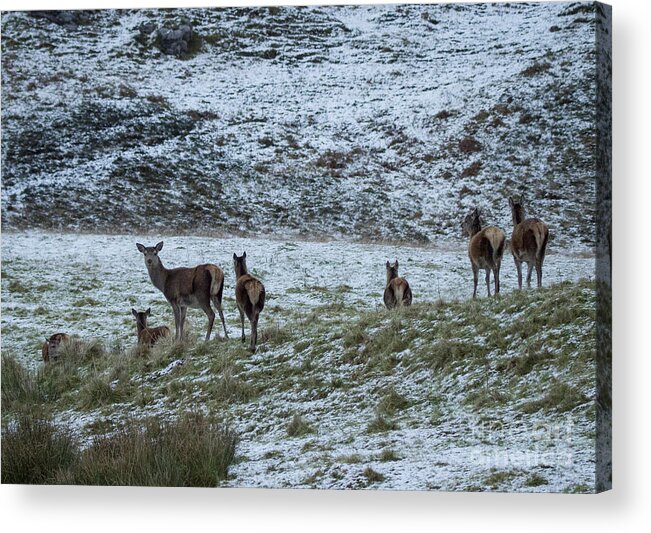The image captures a serene winter scene where a gentle dusting of snow covers a grassy field, suggesting either early winter or a late spring snow. A distinct hill or mountain rises in the background, demarcating the edge where the flat land transitions to an incline. Sparse vegetation, primarily small weeds, dots the snowy terrain, giving an impression of a somewhat barren landscape.

In the foreground stand at least six deer, composed in a natural formation. On the left side, one deer is strikingly facing the camera, its body slightly turned with an ear tilted attentively, showcasing the lighter fur around its eyes. Another deer on this side also appears to be acknowledging the camera. The remaining deer are facing forward, seemingly on their way toward the hill.

The photograph extends around the edges of the canvas, giving it a frameless appearance that fully immerses the viewer in this tranquil outdoor setting. The complete absence of text ensures that the visual narrative remains undisturbed, inviting observers to contemplate the quiet beauty of wildlife in a snowy landscape.